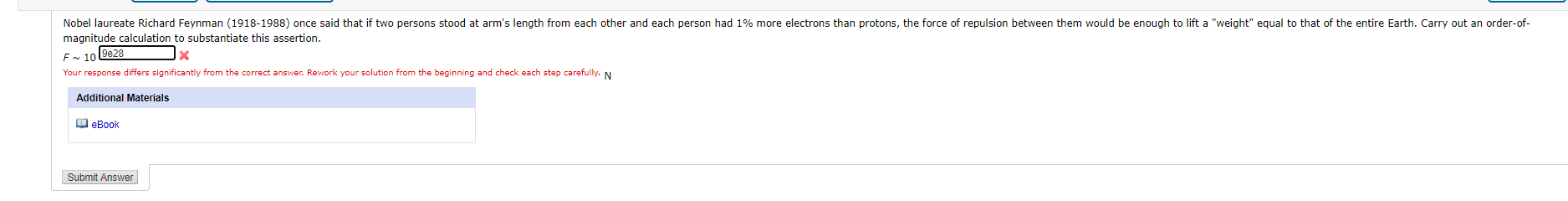This image is a detailed screenshot of a website, which appears to be a quiz interface. The screenshot has a long rectangular shape, with dimensions approximately in a 10:90 height-to-width ratio, portraying the vertical orientation clearly.

At the very top of the image, there is the bottom half of a thin gray bar that spans from left to right. Below this bar, a couple of bluish buttons are partially visible. Directly beneath these buttons, a piece of black text presents a question:

"Nobel laureate Richard Feynman (1918-1988) once said that if two persons stood at arm's length from each other and each person had 1% more electrons than protons, the force of repulsion between them would be sufficient to lift a weight equal to that of the entire Earth. Carry out an order of magnitude calculation to substantiate this assertion."

Following the question, the user's attempted response is displayed. They have written "F > 10" in a text input box, and entered "9e to 8" within the answer field. A red 'X' indicates that this answer is incorrect. Below the input box, a red message reads: "Your response differs significantly from the correct answer. Rework your solution from the beginning and check each step carefully." Next to this message, there's a capital black letter "N."

Underneath this message, the additional resources section is visible. A box with a blue top contains the label "Additional Materials" in black text, and beneath it, a blue hyperlink directs to an e-book.

Finally, at the bottom left-hand corner of the image, a gray button labeled "Submit Answer" is present, which suggests the user can submit or resubmit their answer after re-evaluation.